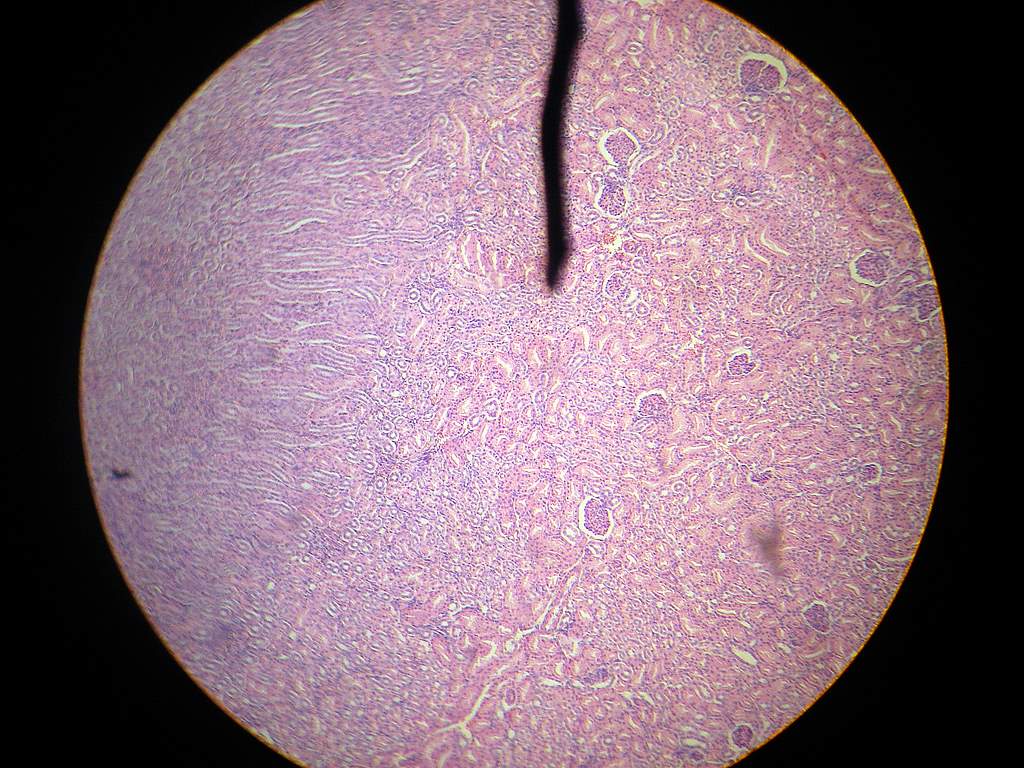The image depicts a centrally located large circular sphere set against a completely black background. The sphere displays a blend of light pink and purples, resembling a detailed pattern that could be seen under a microscope. It features various dark purple circular sections, interspersed with wavier white lines on the left side and scattered white spots toward the bottom, giving it an amoeba-like appearance. Intriguingly, a single black line descends from the top center through the middle of the sphere, potentially indicating a shadow or a crack. The image lacks any text, emphasizing its complex texture and coloration. The design within the sphere showcases intricate squiggles and patterns, primarily purple with accents of dark purple and white, possibly hinting at a scientific slide view of microorganisms or bacteria. This overhead perspective enhances the impression of observing a biological specimen in detail.